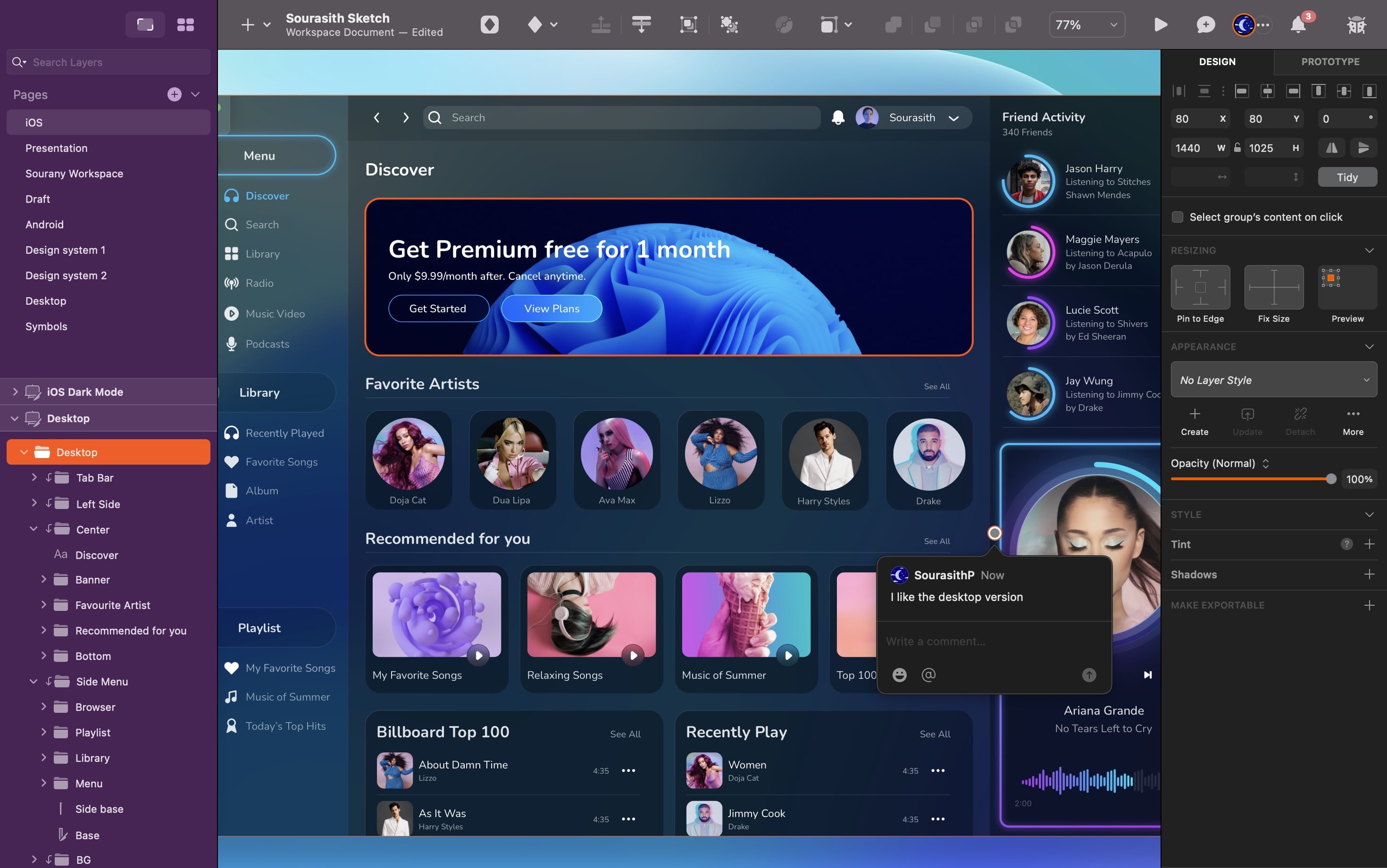The image depicts a webpage, seemingly part of a design or content management system, with multiple interface elements and navigation options. On the left side, there is a detailed menu bar that includes options like "Search Layers," "Pages," "iOS Presentations," "Sorany Workspace," "Draft," "Android," "Design System 1," "Design System 2," and "Desktop Symbols." 

In the middle section, there are two highlighted tabs: one with a lighter purple color labeled "iOS Dark Mode," and another simply labeled "Desktop." An orange drop-down menu labeled "Desktop" also appears prominently. Beneath these elements, there is a series of navigation options: "Tab Bar," "Left Side," "Center," "Discover," "Banner," "Favorite Artists," "Recommended for You," "Bottom," "Side Menu," "Browser," "Playlist," "Library," "Menu," "Side Base," and "Base."

At the top of the page, there are several interface elements including the text "Sourasith Sketch Workplace Document Edited." Additionally, there is a tool dropdown menu showing "77%," three notifications, and promotional content offering a premium subscription with the text "Get Premium for one month free, only $9.99 a month thereafter, cancel anytime," followed by "Get Started" and "View Plans" buttons.

On the left side of this central area, another menu is visible with options for "Menu," "Discover," "Search," "Library," "Radio," "Music," "Videos," "Podcast," and "Recently Played." This comprehensive layout seems to be aimed at organizing and navigating through various digital assets and design elements efficiently.